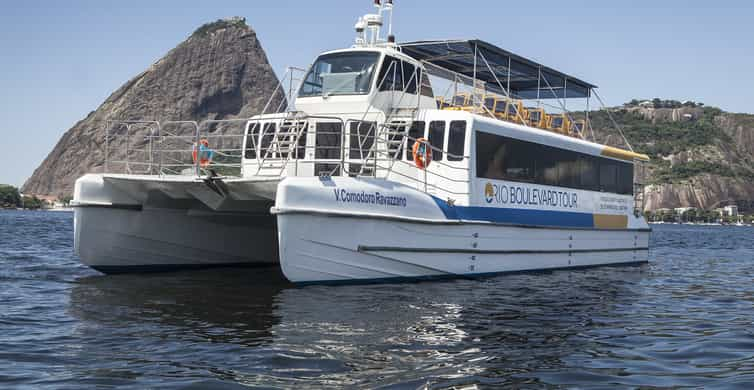A detailed photograph captures a sizable white catamaran boat called "Rio Boulevard Tour" gliding over dark blue waters under a clear blue sky. The catamaran, designed for tours, showcases distinctive twin pontoons and features an expansive indoor area with dark glass windows on the lower deck. Above, the open upper deck with a sunroof offers ample seating, capable of hosting 30 to 40 people. The boat also sports blue and tan lines on its hull. Markings on one side of the boat read "V Commando Ravezero" or "W Commodoro Rabazzano." In the background, massive gray rock formations dominate the left side, while to the right, a seaside landscape with green vegetation and rocky cliffs enhances the scenic view. The image exudes a sense of leisurely exploration and the natural beauty surrounding the chartered excursion.